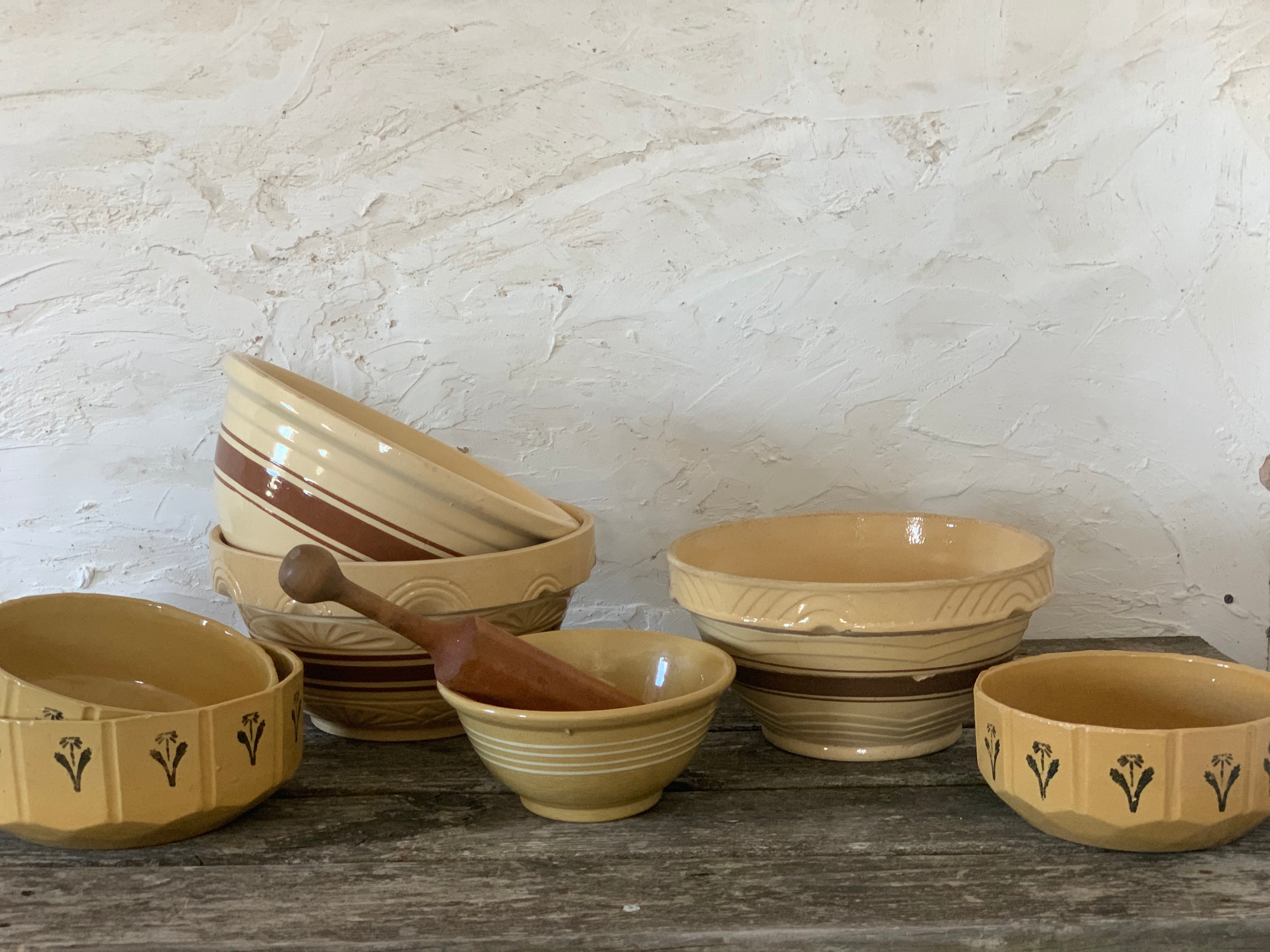The photograph captures a collection of seven terra cotta bowls arranged haphazardly on a worn, brown, planked wooden table against a rough, cream-colored stucco wall. The bowls vary in size, shape, and texture. On the left, two smaller terracotta bowls adorned with black floral patterns nest inside one another. To their right, a larger bowl with a brown stripe around the outside contains another smaller bowl. At the table's center, a small light terracotta bowl features a wooden tool that appears to be for mashing, possibly for cornmeal. To the right of this, there is another large striped bowl with intricate squiggly lines engraved upon it, and on the far right is a round bowl with matching floral designs. The overall arrangement and the aged, rustic elements of the table and backdrop give the scene a timeless, artisanal quality.